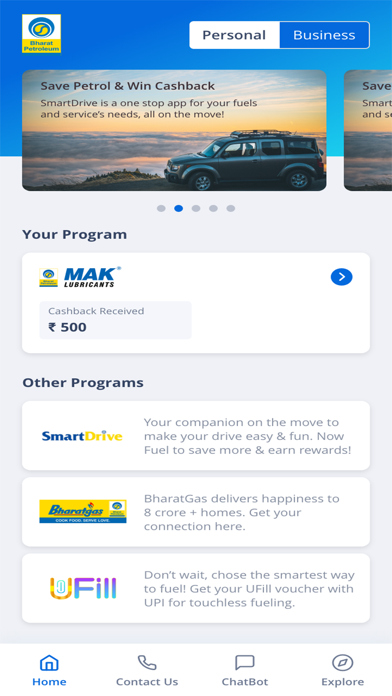Here is a cleaned-up and detailed caption for the image described:

---

The image showcases a website header with a prominent blue banner that transitions from a darker blue at the top to a lighter blue toward the bottom. At the very top, a square icon is displayed along with the text "Barrett Petroleum" (spelled B-H-A-R-A-T). Below this, there are two links: "Personal" in white text on a blue background, and "Business" in blue text on a white background.

A visually engaging outdoor scene is featured with the slogan "Save Petrol and Win Cash Back" overlaying the sky. Just beneath this, there's a promotional message that reads: "Smart Drive is a one-stop app for your fuel and service needs, all on the move."

Moving further down, the background turns light gray, displaying a banner that announces "$500 Cashback Received" for "Mac Lubricants." Above this banner, the text "Your Program" is prominently displayed.

Continuing down the page, three separate banners under the section "Other Programs" are visible. The first banner, showing "Smart Drive," features "Smart" in blue text and "Drive" in yellow text. Adjacent to it are banners for "Barrett Gas" and "UFIL."

At the very bottom of the page, there is a navigation section with options labeled "Home" in blue font, along with "Contact Us," "Chat Box," and "Explore."